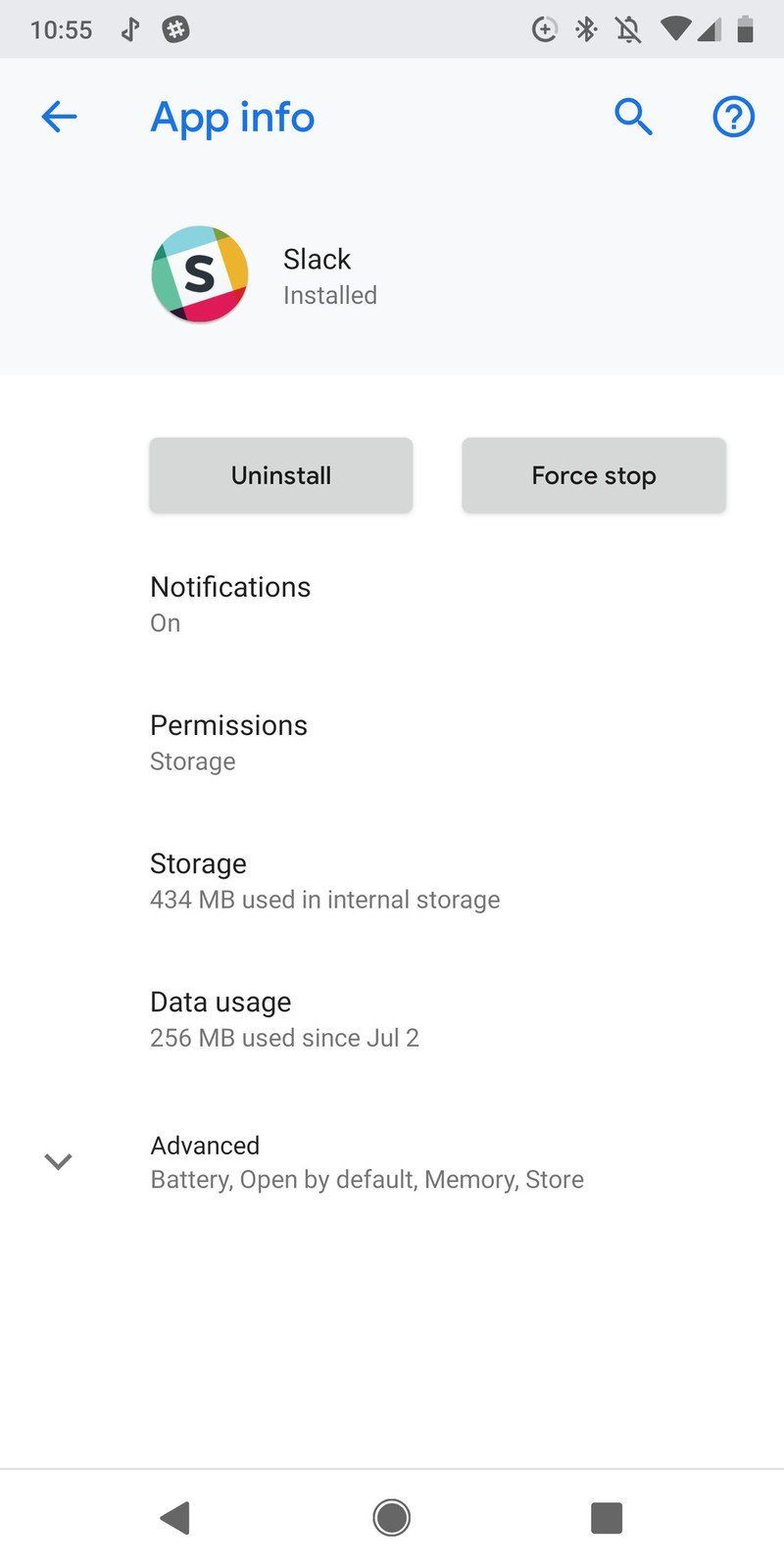In this image, we observe a screenshot of a mobile device. The top-left corner displays the current time, which is 10:55. In the top-right corner, several status icons are present: the data saver icon, Bluetooth connected icon, Do Not Disturb icon, WiFi signal icon, network signal bar, and battery bar. Below the status bar, the main content of the screen shows detailed information about an application. The interface includes options for "App Info" and a search icon. The app in question is Slack, with options to "Uninstall" or "Force Stop" the application. Notifications for Slack are turned on. Additional sections include "Permissions," "Storage," and specific details such as "Storage: 434 MB used" and "Internal Storage: Data."